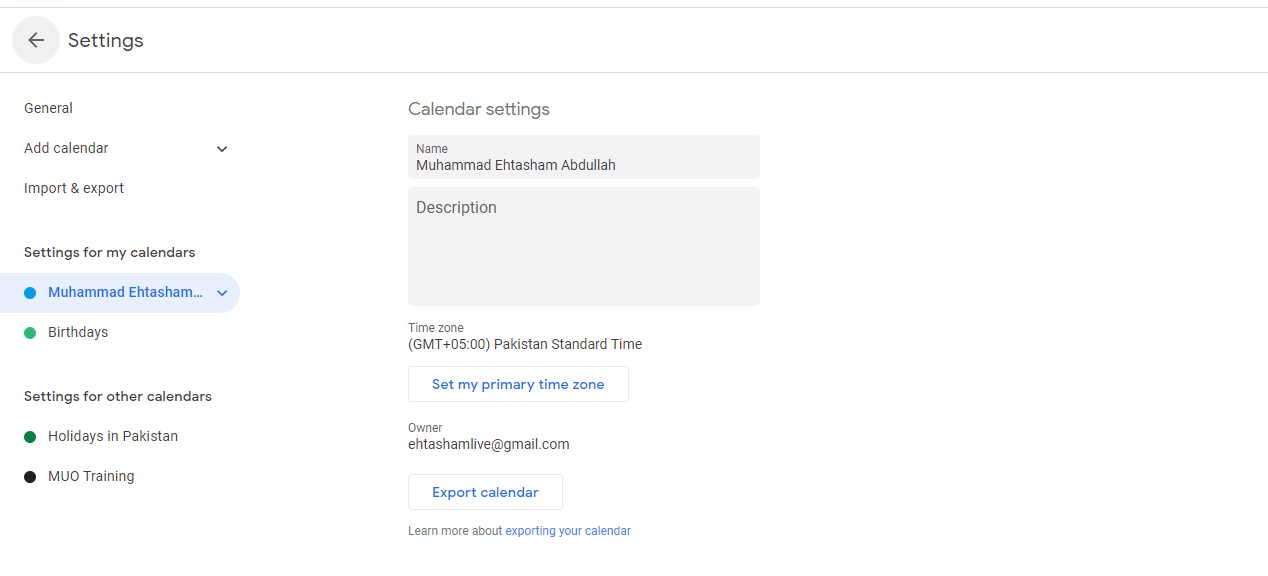Here's a polished and detailed caption for the image:

---

**Website Control Interface Screenshot**

The screenshot captures a control interface for a calendar management section of a website. The layout is primarily white with black font, providing a clean and simple design. In the upper left corner, there is a left-pointing arrow labeled "Settings." Below this, the options listed include "General," "Add Calendar" (with a downward arrow), and "Import & Export."

Further down, the interface is divided into sections. The first section, titled "Settings for my calendar," features a teal dot accompanying the name "Muhammad Estasam," and a green dot for "Birthdays." 

The next section, "Settings for other calendars," contains a green dot corresponding to "Holidays in Pakistan" and a black dot labeled "MUO Training."

On the right side of the screen, the "Calendar Settings" section includes fields for "Name" and "Description," the latter of which is currently blank. The "Name" field displays "Muhammad Estasam Abdullah." Directly beneath, the time zone is designated as "GMT +5:00 Pakistan Standard Time," with a blue button labeled "Set my primary time zone" positioned below. Further down, owner details are provided with the email address "estahemlive@gmail.com." A blue link titled "Export Calendar" is present, and underneath it, in smaller font, the text "Learn more about exporting your calendar" is available, with "Exporting your calendar" also being a clickable link.

The interface boasts a symmetrical, user-friendly design, making it straightforward and easy to navigate.

---